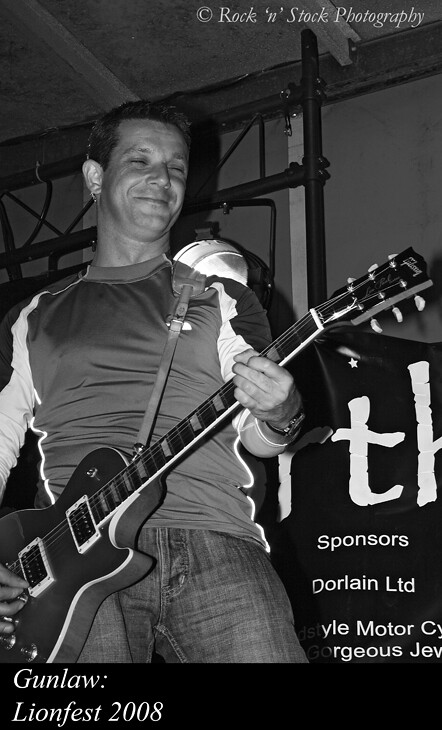This detailed black-and-white photograph captures a joyful moment of a Caucasian man, likely in his 30s or 40s, playing an electric guitar on stage, indoors in a concert hall or bar setting. He is dressed in blue jeans and a long-sleeved shirt, with a watch on his left wrist. His eyes are closed and he has a content, closed-mouth smile, looking downward at his instrument. The backdrop behind him, filled with ceiling rigging and black pipework, features a partially visible banner displaying sponsors such as "D.O.R.L.A.I.N. Limited" and other fragmented names like "V.I.E. V.L.E. Motor" and "R.G.E.O.S. J.E.V." Text on the photograph reads at the top, "Copyright Rock and Stock Photography," while the bottom left states, "Gun Law: Lion Fest 2008."